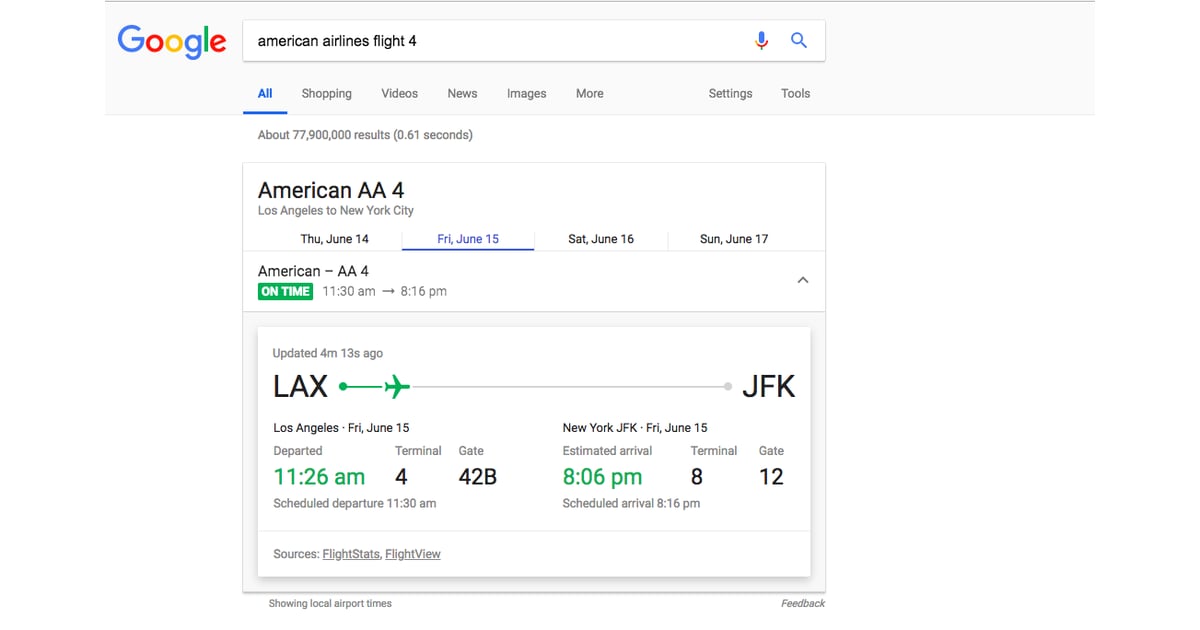The screenshot depicts a Google search results page for "American Airlines flight 4." In the top left corner, the iconic Google logo is visible, indicating that the search was conducted using Google. Adjacent to the logo is the search bar containing the query "American Airlines flight 4." Below the search bar, the blue-highlighted "All" tab shows the active search category. To the right of this tab are additional categories including "Shopping," "Videos," "News," "Images," and "More," followed by "Settings" and "Tools" options situated on the far right.

The search results reveal approximately 77,900,000 results. The primary result displayed is for "American Airlines flight 4" (AA4), detailing a flight from Los Angeles to New York City. Multiple date options are listed beneath this result: Thursday, June 14th, Friday, June 15th, Saturday, June 16th, and Sunday, June 17th. The highlighted date is Friday, June 15th.

Further details for the selected date show that the flight, AA4, is reported to be on time, scheduled from 11:30 AM to 5:15 PM or 8:15 PM. Below these details, a progress bar illustrates the flight's status relative to its departure and arrival points at JFK airport.